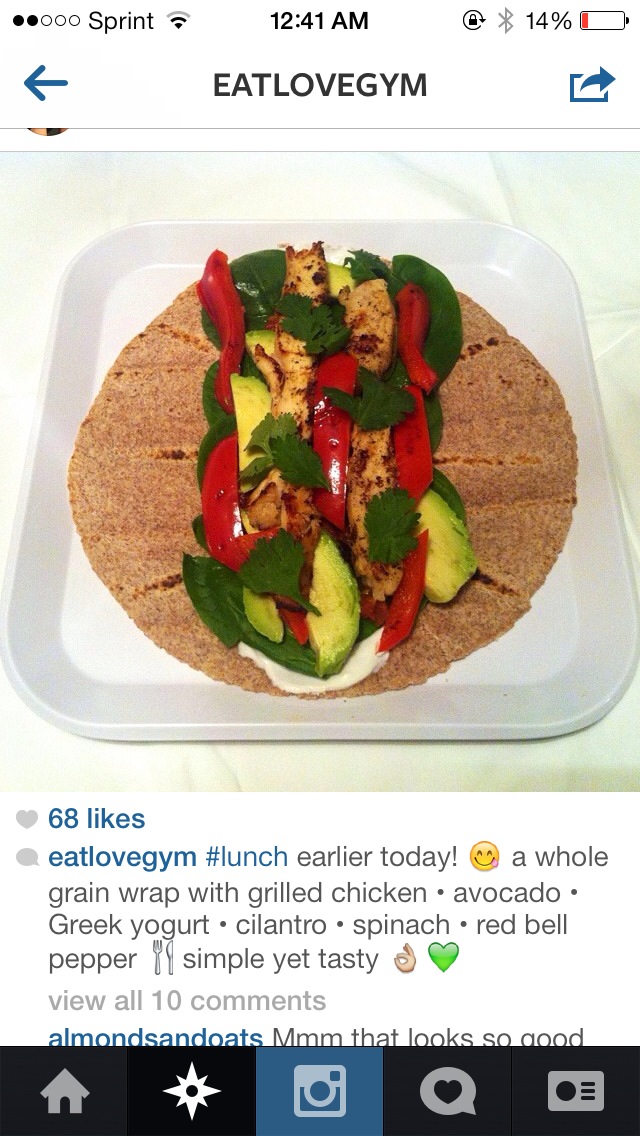This social media post from EatLoveJim features a mouth-watering photo, captured as a screenshot on a cell phone displaying Sprint as the service provider, with a 14% battery at 12:41 AM. The post showcases a delicious whole grain wrap on a white square plate. The wrap is filled with grilled chicken, avocado, Greek yogurt, cilantro, spinach, and red bell peppers. The caption reads: "Hashtag lunch earlier today, simple yet tasty," accompanied by a fork and knife emoji, a smiley face emoji, a peace sign, and a green heart. The post has garnered 68 likes and invites engagement with a prompt to view all 10 comments. The image captures an enticing and healthy meal, highlighting its simplicity and deliciousness.